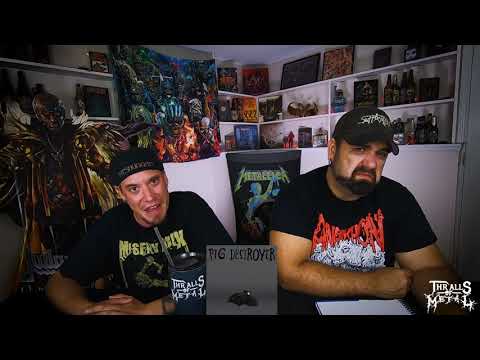This image appears to be a screenshot from a YouTube video or channel, likely centered around metal music. In the frame, two middle-aged men, possibly in their 40s or 50s, are sitting at a table with a black tablecloth. Each man is wearing a black t-shirt and a black ball cap. The man on the left has a backward-facing hat and a black shirt featuring lime green elements, with the phrase "Pig Destroyer" on it. The man on the right, with a forward-facing hat, has a black t-shirt with red and white screen print.

On the table between them, there's a sign with a gray background that also reads "Pig Destroyer." In front of the man on the left sits a cup, and there may also be a notebook present. Behind them, the room's walls are mostly white with various decorations, including a prominent Metallica poster, other artistic portraits, and shelving that holds glass bottles and figurines. Additionally, there is a cardboard cutout stand-up of a video game character on the left side of the image.

Both men look like they are either reviewing or discussing metal music, evidenced by the logo "Thralls of Metal" seen in the bottom right corner of the image. They appear to be engaged in a detailed content session likely for YouTube, capturing the essence of their shared interest in the genre.